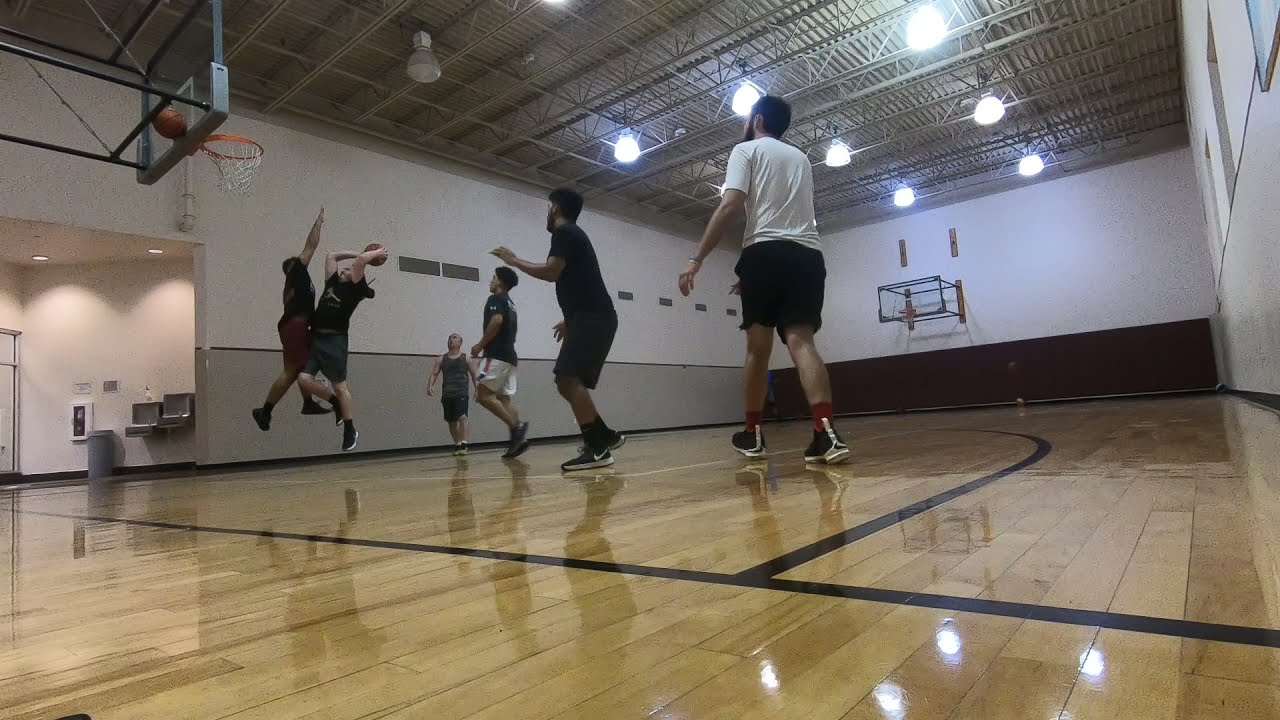In this image, we see the inside of a gleaming gymnasium with a full-sized basketball court, flanked by nets on both ends. The court floor is impeccably polished, reflecting the overhead lights, although two lights nearest the basketball net are not functioning. The walls of the gym contrast, with the back wall featuring a maroon or brown lower section beneath the basketball goal and white above, while the side wall near the entrance is grayish off-white on the bottom and white on top. 

In the top left corner of the image, metal bars are visible, which support the elevated basketball hoop. Six young men are engaged in a game: on the left side, a defender has both hands raised and is airborne, attempting to block a shot from an opposing player who is also in mid-air. Meanwhile, on the right side of the court, another four players are either preparing for a rebound or observing the play, with one noticeably wearing a white shirt and black shorts, and another appearing to be slowly moving towards the action. A basketball can be seen stuck behind one of the nets.

Just outside the entrance to the gymnasium, there is a trash can, a fire extinguisher, and two water fountains, though the view beyond this point is obscured. The overall scene suggests a newly constructed facility with no visible scuff marks on the court floor.